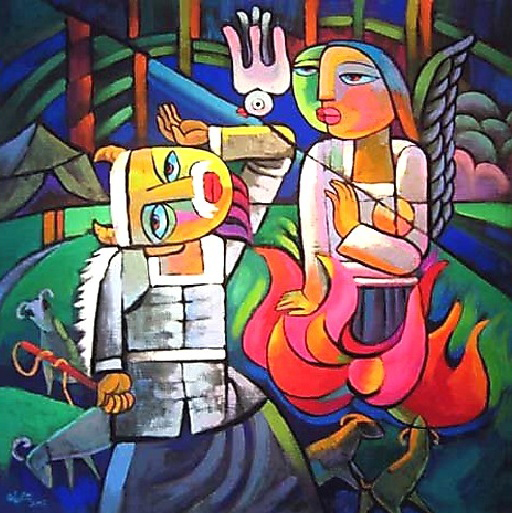The painting is a vivid, stained glass-style artistic rendering featuring two central figures against a colorful backdrop of trees and sky dominated by hues of blue, green, and red. The person on the right, depicted as a silver-suited man with a white mustache, red lips, and golden horns, is dramatically cocking his head to the right. His attire includes a fur cape, and he holds up one hand while the other hangs by his side. He appears to be engaged in a dance, wielding a stick with a serpent coiled around it. On the left stands a woman in a white shirt with striking black wings, from beneath whose skirt emanates vibrant flames in a medley of red, yellow, and orange. Alongside this fiery display are two goats and two small dogs positioned near the front of the image. Dominating the central upper portion of the painting is a white dove, captured mid-dive towards the ground. The overall scene is imbued with an abstract, ethereal quality underscored by its stained glass aesthetic and the rich, interwoven colors of the composition.